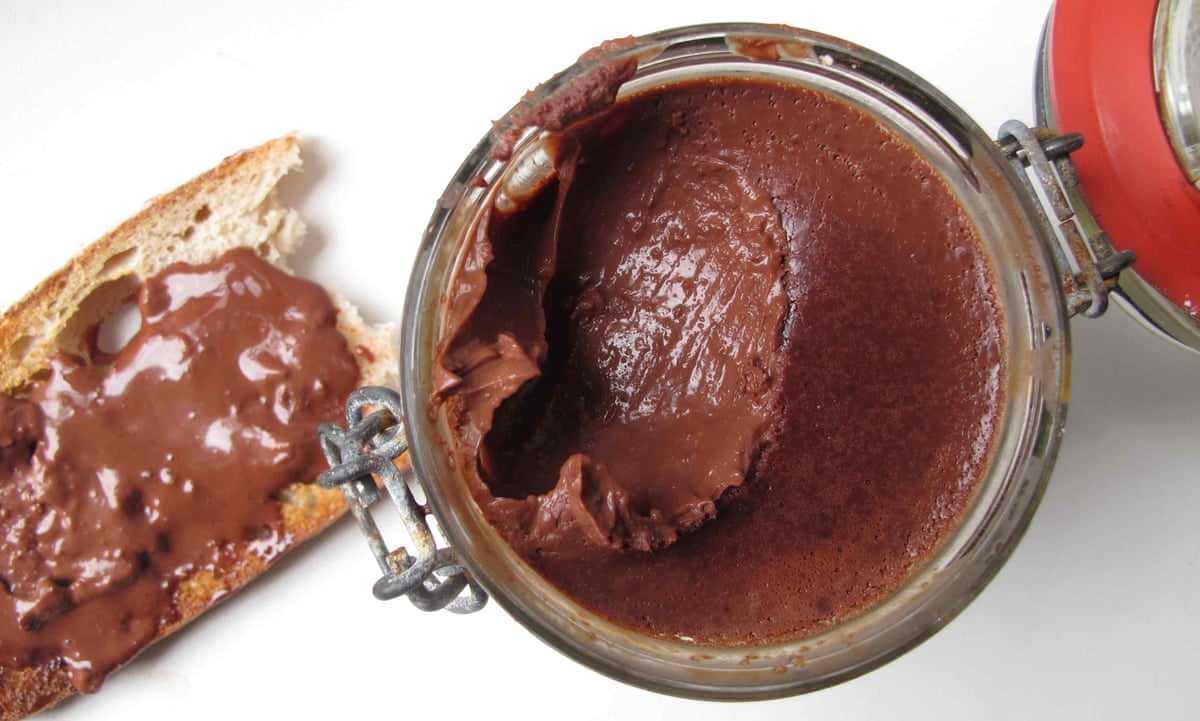The image captures a top-down view focusing on a homemade hazelnut spread or possibly chocolate spread, housed in a jar that occupies about half of the frame. The jar, with a red rubber stopper and a clip-sealing lid, contains a dark brown spread, richer in color than regular peanut butter. A generous scoop has already been taken from the middle, leaving some of the spread around the rim. To the left of the jar, there is a piece of white bread with a portion of the spread already applied and looking enticing, as if recently bitten into. The scene is set against a plain white surface, emphasizing the brown, tan, red, and silver hues of the objects.